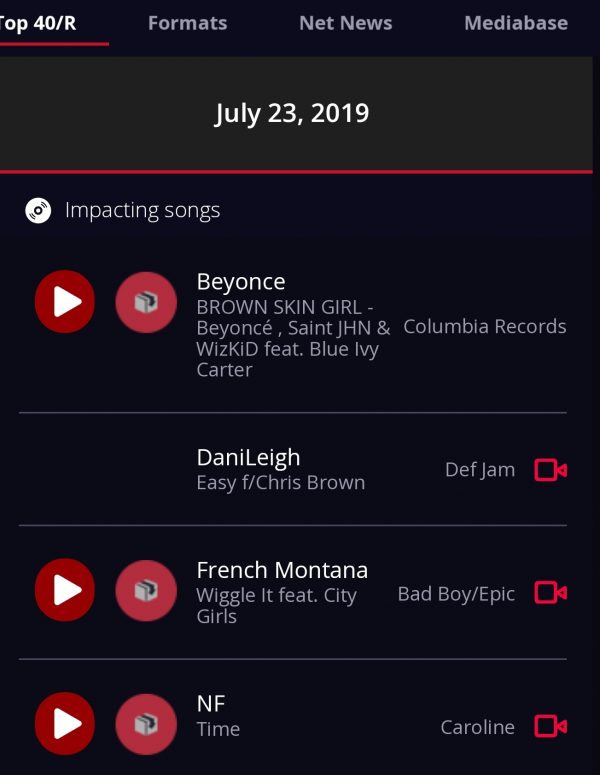**Screen Capture Description: Top 40/R Impacting Songs on July 23, 2019**

The image is a screen capture of a portion of a web page showcasing a music chart from July 23, 2019. At the top, in the upper ribbon section, there are several menu options displayed horizontally: "Top 40/R", "Formats", "Net News", and "Mediabase". A distinct red horizontal line underscores the "Top 40/R" label.

Directly below this ribbon, the date "July 23, 2019" is clearly printed, with "July" spelled out. Another thin red horizontal line is present under the date line. Below these elements, the main content is organized horizontally into several segments.

The first item in this section is a play button icon for audio playback. Next to it, there is a circular icon that resembles a small toaster or similar object. The title "Beyoncé - Brown Skin Girl" follows this, indicating the song "Brown Skin Girl" by Beyoncé featuring SAINt JHN, Wizkid, and Blue Ivy Carter, under Columbia Records.

Following the Beyoncé entry, details of another song are displayed: "DaniLeigh - Easy" featuring Chris Brown, listed under Def Jam Recordings.

Further to the right, two additional artists are mentioned: French Montana and NF, suggesting their songs are also featured on the impacting songs playlist for that date. 

The entire layout signifies a segment of impactful songs that were noteworthy on this specific date, providing a snapshot of popular music tracks within the Top 40/R genre.